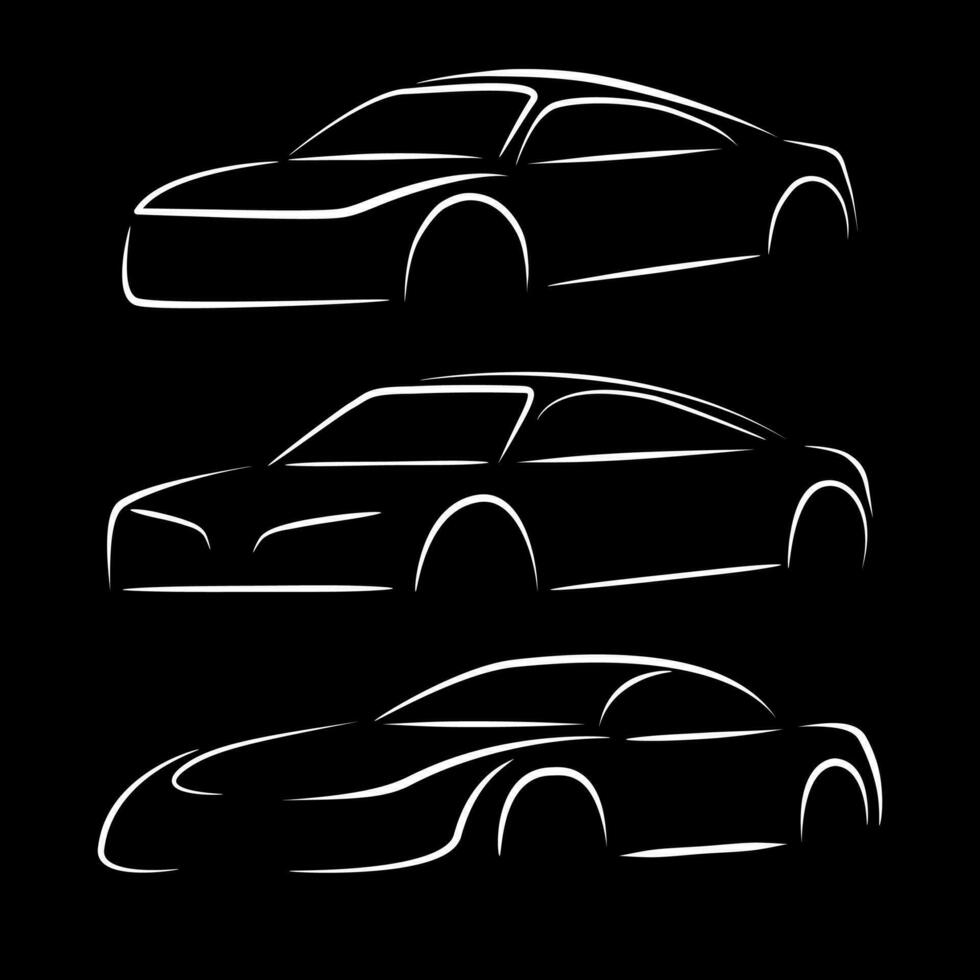The image features a minimalistic graphic that resembles a logo. Set against a completely black background, three white line drawings depict different car models, arranged vertically. The top car is a boxy, small four-door sedan, presented with an outline that excludes detailed features like doors or wheels. The middle car, while similar in shape to the first, has a more aerodynamic design with a sleeker hood. The bottom car, exuding a designer feel, features smoother lines and a more refined roof and front end, suggesting a sporty, high-end vehicle. The white lines are thick and do not connect fully, offering a stark contrast against the black background and highlighting the essential contours of each car.